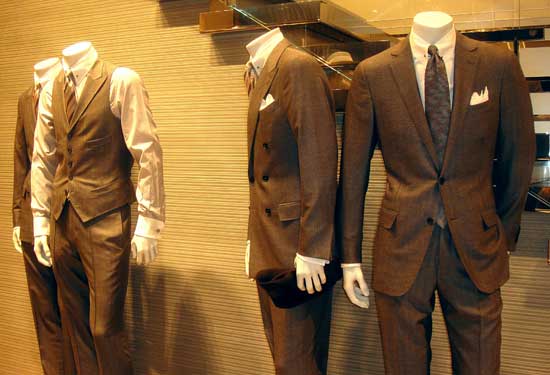In this detailed image from a storefront showcasing men's suits, we see four headless mannequins, each meticulously dressed in various styles of formal wear. The mannequins are positioned against a beige-colored wall with fine horizontal striping, next to a staircase with a glass railing leading to the upper part of the store. 

The mannequins display an array of sophisticated outfits. Starting from the left, the first mannequin flaunts a full suit complete with a long-sleeved white collared shirt, a brownish tie, a suit coat with buttons, and matching pants. A white handkerchief peeks out from the front left pocket of the coat. Next to it stands another mannequin, slightly turned to the side, dressed in a white long-sleeve button-down shirt paired with a grayish-brown vest fastened with four buttons and finished off with matching pants. This mannequin’s sharp ensemble is complemented by cufflinks.

In the background, the third mannequin features a suit with a suit coat displaying three buttons, a white collared shirt, and another pocket handkerchief. This mannequin's attire also seems brown-tinted, possibly due to the lighting. The final figure, positioned at a slight angle, reveals parts of a suit coat and pants that mirror the brownish-tan hue seen in others.

The overall display is carefully arranged to highlight different styles including double-breasted and single-button suits, as well as various accessories like handkerchiefs and ties, catering to an elegant and refined male wardrobe.